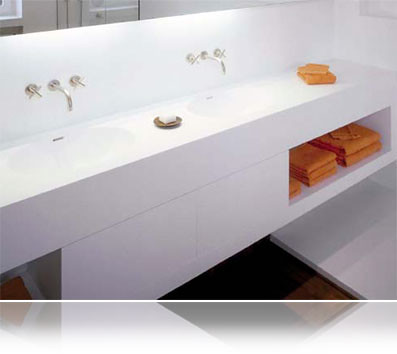This photograph depicts a stylish and modern bathroom, likely situated in a home or upscale hotel. The centerpiece of the image is the flat, white countertop, which seamlessly extends into the front of the cabinets below, creating a sleek and cohesive design. The countertop houses two inset white ceramic sinks, providing a clean and flush appearance.

To the far right of the counter, two neatly folded, vibrant orange towels are stacked atop each other, adding a pop of color to the otherwise neutral palette. Near the center of the countertop sits a brown coaster holding a pristine white bar of soap, subtly highlighting the attention to detail in the decor.

The faucets, mounted on the white back wall above the sinks, feature an elegant design with outward-extending spouts that droop downwards into the sinks. Each faucet is flanked by cross-designed dials, offering both functionality and an extra touch of sophistication. Just above the faucets, a glimpse of a mirror can be seen, hinting at the mirrored wall likely spanning the length of the countertop.

Beneath the countertop, there are two white cabinet drawers without visible knobs, emphasizing a minimalist aesthetic. An open shelf below them showcases an organized stack of orange towels: a set of two towels next to a set of three, further contributing to the room's meticulously curated look.